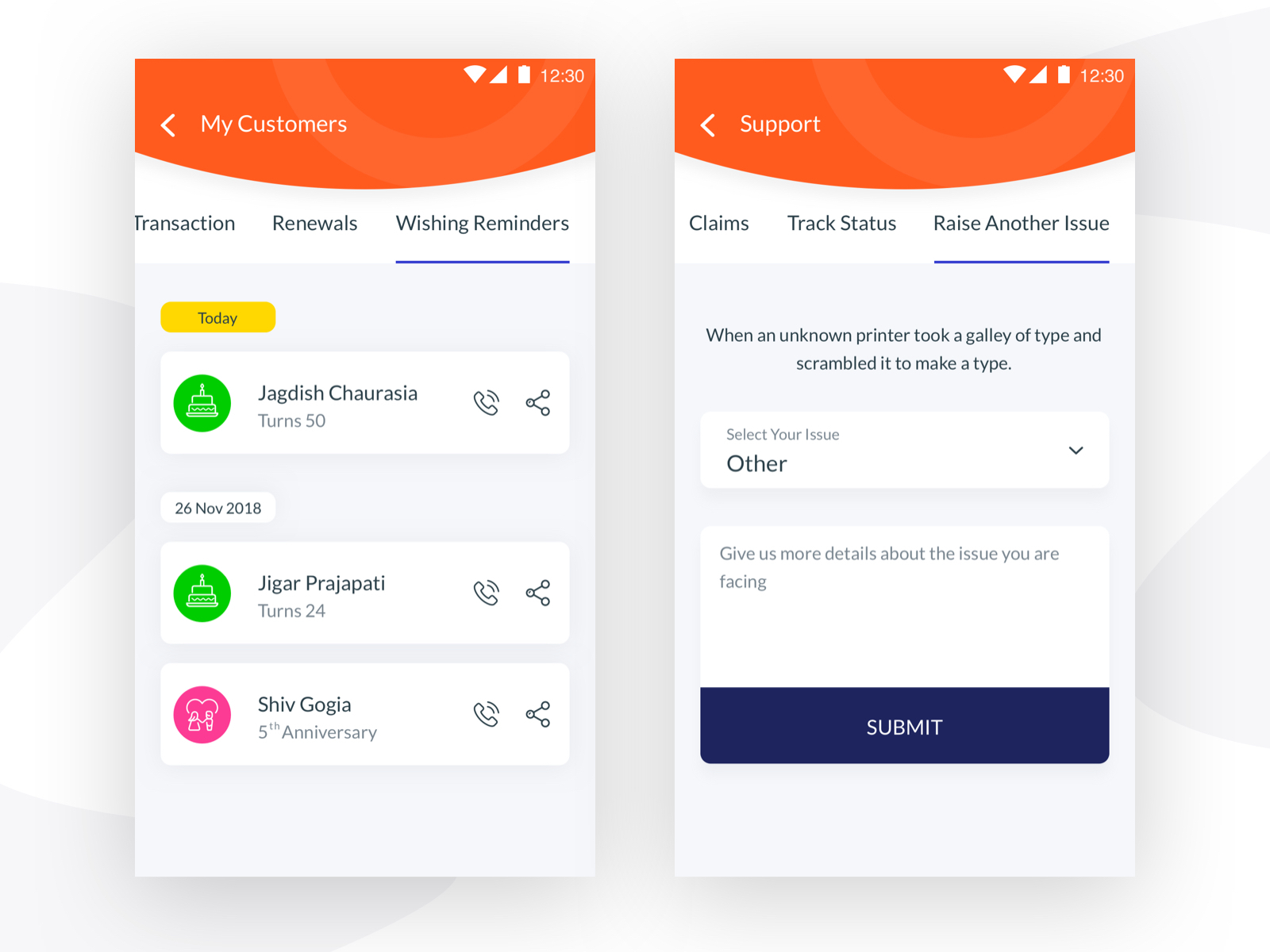This image displays two pages on a cell phone screen, showcasing the time as 12:30. Both pages feature orange headers with a semi-circular shading design, giving them a distinctive, scalloped bottom edge.

On the first page, the header contains the text "My Customers" in white. Below the orange header is a white background with several segmented sections: 
- The first section lists "Transaction Renewals" and "Wishing Reminders," with "Wishing Reminders" underlined in blue. 
- Under the gold bar labeled "Today," there are entries for Jagdish Chershia and Jagar Prajapati, each accompanied by green circles, a phone icon, and an internet connection icon. The date "26 November 2018" is also mentioned.
- Further down, a white box highlights a pink circle with "Shiv Gorgia 5th anniversary," along with the same phone and internet connection icons.

The second page's orange header reads "Support" in white text. Below it, the white background contains options: "Claims," "Track Status," and "Raise Another Issue" with the latter underlined in blue. In the gray section below, placeholder text reads, "When an unknown printer took a galley of type and scrambled it to make a type." Further instructions prompt the user to "Select your issue" and provide more details in the text area labeled, "Give us more details about the issue you are facing." At the bottom of this form is a blue "Submit" button.